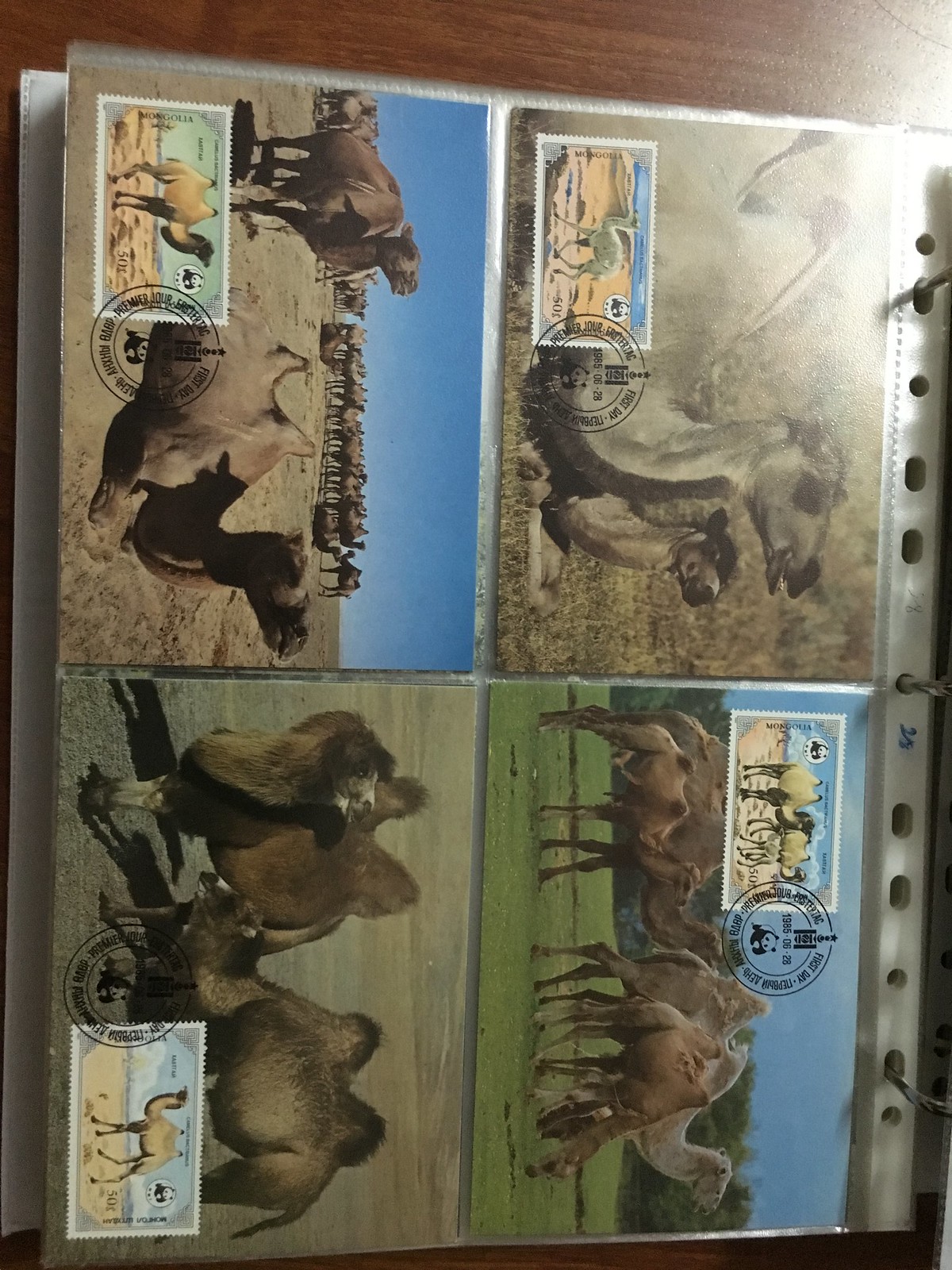This is a photograph of four camel-themed postcards laid side by side within a clear plastic file in a three-ring binder, visible from the left-hand side of the image. The binder appears to be sitting on a wooden table, and the postcards are rotated slightly clockwise, making them appear sideways. Each postcard features a distinctive scene with camels as the main subject, and all have postal stamps depicting camels.

The top left postcard depicts two camels in the foreground amidst a herd of camels in the background under a blue sky. The top right postcard shows an adult and a baby camel standing in a greenish-brown grassy area. The postcard below it features several adult camels and a baby camel on green grass with trees and a blue sky in the background. The bottom left postcard is a close-up of two camels standing in dark green grass. Each postcard includes a detailed camel stamp, with the stamps varying slightly in position but consistently showcasing camels on sandy ground under a blue sky.